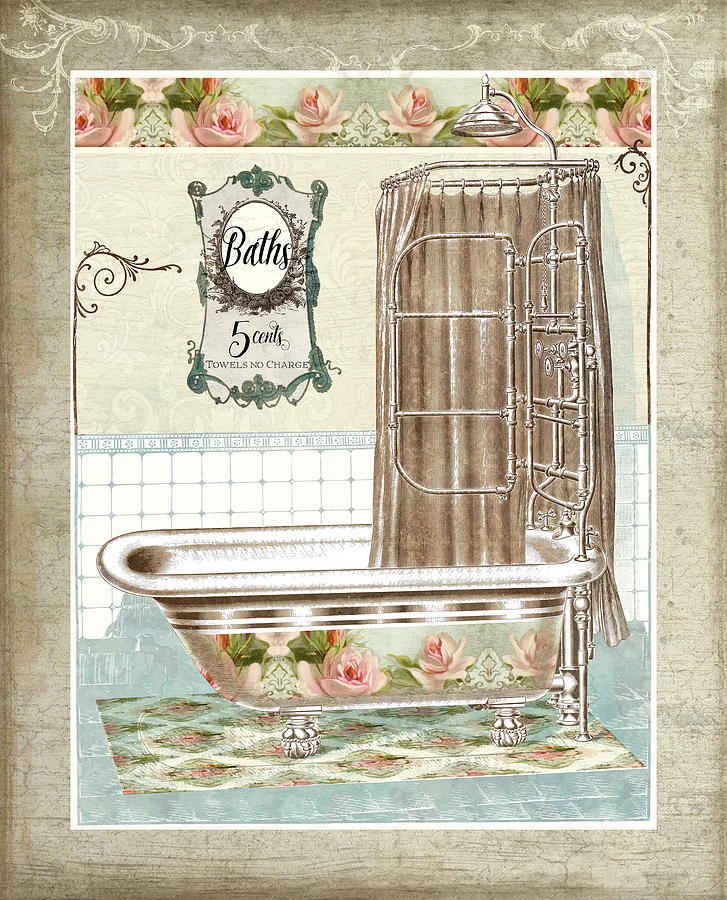This image features an elegant, vintage-inspired wall art print, ideal for bathroom decor. The piece showcases a central illustration of a Victorian-style bathroom with a prominent clawfoot bathtub adorned with pale pink cabbage roses. The tub rests on a teal floor and is accompanied by a partially visible brown shower curtain and an overhead showerhead extending toward the floral border. Surrounding the main image is a tan, wood-grain-like frame with intricate, scalloped, vine-like detailing at the top, imparting a weathered and antique charm.

Above the bathtub, the wall is decorated with a vintage beige wallpaper, complete with a white scalloped border featuring delicate scrolling designs and pink cabbage roses. A sign on the wall humorously reads, "Baths. Five cents. Towels. No charge." The background includes the lower portion of the wall in white tile, adding to the historical aesthetic. The overall style and details evoke a Victorian ambiance, making it a unique and detailed piece for a nostalgic bathroom setting.